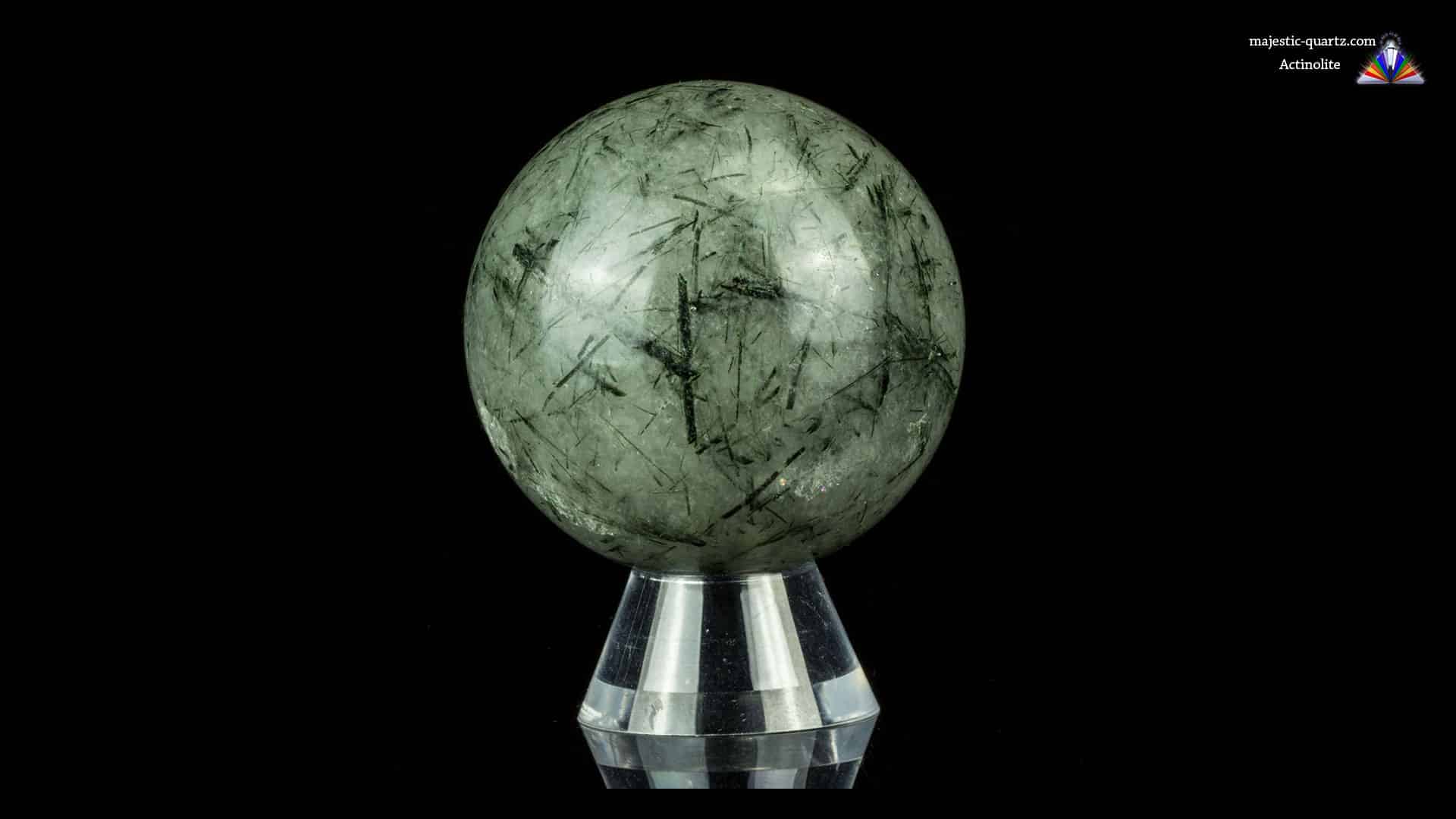The image features a polished, light green crystal sphere, displaying intricate, dark green patterns that resemble crow's feet, forming Y or X shapes throughout the stone. The sphere is finely cut, sanded, and polished, resulting in a shiny surface that reflects light. It is mounted on a discreet, clear stand, designed not to distract from the crystal's beauty, and set against a plain black background to prominently highlight the intricate details and vibrant color of the crystal. The photograph additionally includes a logo and website for MajesticQuartz.com in the upper right corner, although the specific name of the crystal, comprised of text beginning with an 'A', is too small to discern.